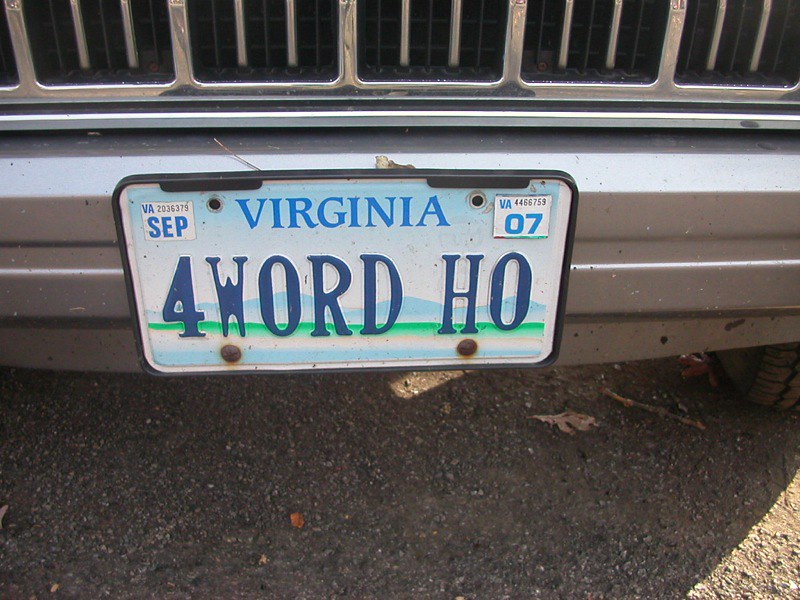This detailed image captures the front of a vehicle, which could possibly be a car or truck based on the partial grill that is visible. The vehicle has a chrome bumper with chrome grill work above it. The main focus of the image is the Virginia license plate, prominently displaying "4WORD HO" in blue text. The plate features distinctive Virginia scenery, including a blue sky, darker blue mountains halfway up the plate, a green line, and a cream-colored stripe across the bottom. Two bolts secure the plate at the bottom, while the top lacks any bolts. In the top left corner of the license plate, there's a September sticker with small numbers above it, and in the top right corner, a 2007 sticker with "VA" in blue letters. The license plate is set in a solid black holder without any frame. The vehicle is parked on gravel, illuminated by sunlight visible beneath it, accentuating the overall nostalgic feel of the scene while indicating the year and month of the registration tags.